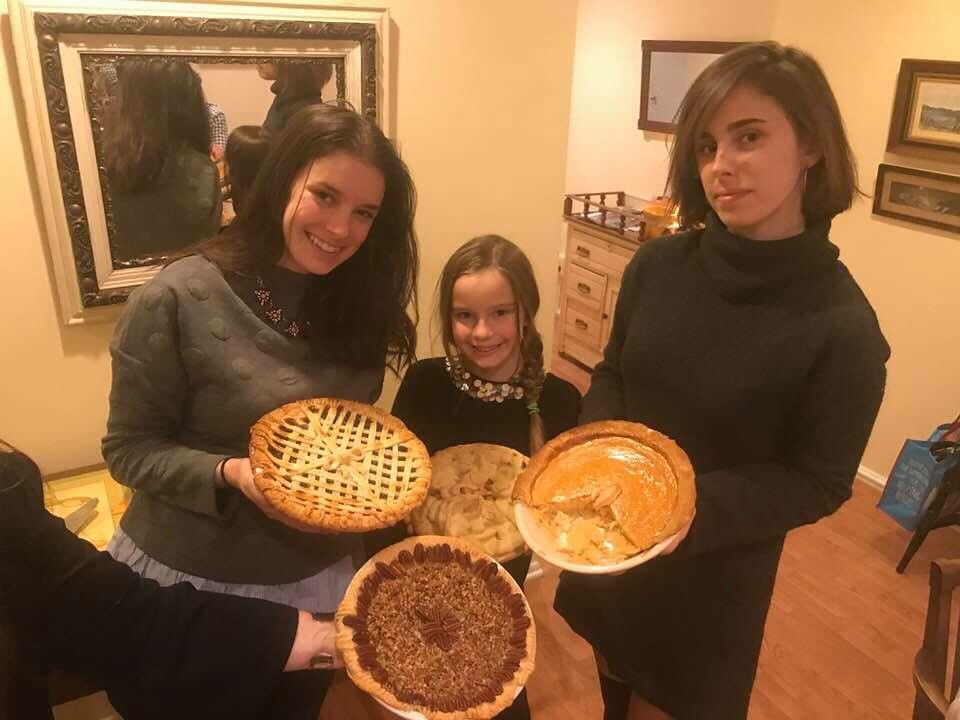In the well-lit room of a cozy home, three family members—two women and a little girl—stand at the center of the photograph, each holding up a homemade pie and smiling warmly at the camera. To the left stands a young woman in her 30s with long, dark hair parted in the center. She has light skin and is dressed in a black top beneath a gray sweater adorned with embossed circles, holding a lattice-top pie and leaning slightly to her left. In the middle, a little girl with blonde hair styled in a braid and parted slightly off-center holds her pie confidently. On the right is a teenager or a woman in her early 20s, with straight, dark brown hair just above her shoulders and parted on the right. She wears a dark green turtleneck sweater and tilts her head to the left while looking upward. An arm extending from the photo's lower left corner, clad in a black sleeve, holds a large pecan pie front and center. Behind them, adornments such as a mirror, framed pictures on cream-colored walls, and a light brown cabinet add a homely touch to the setting.